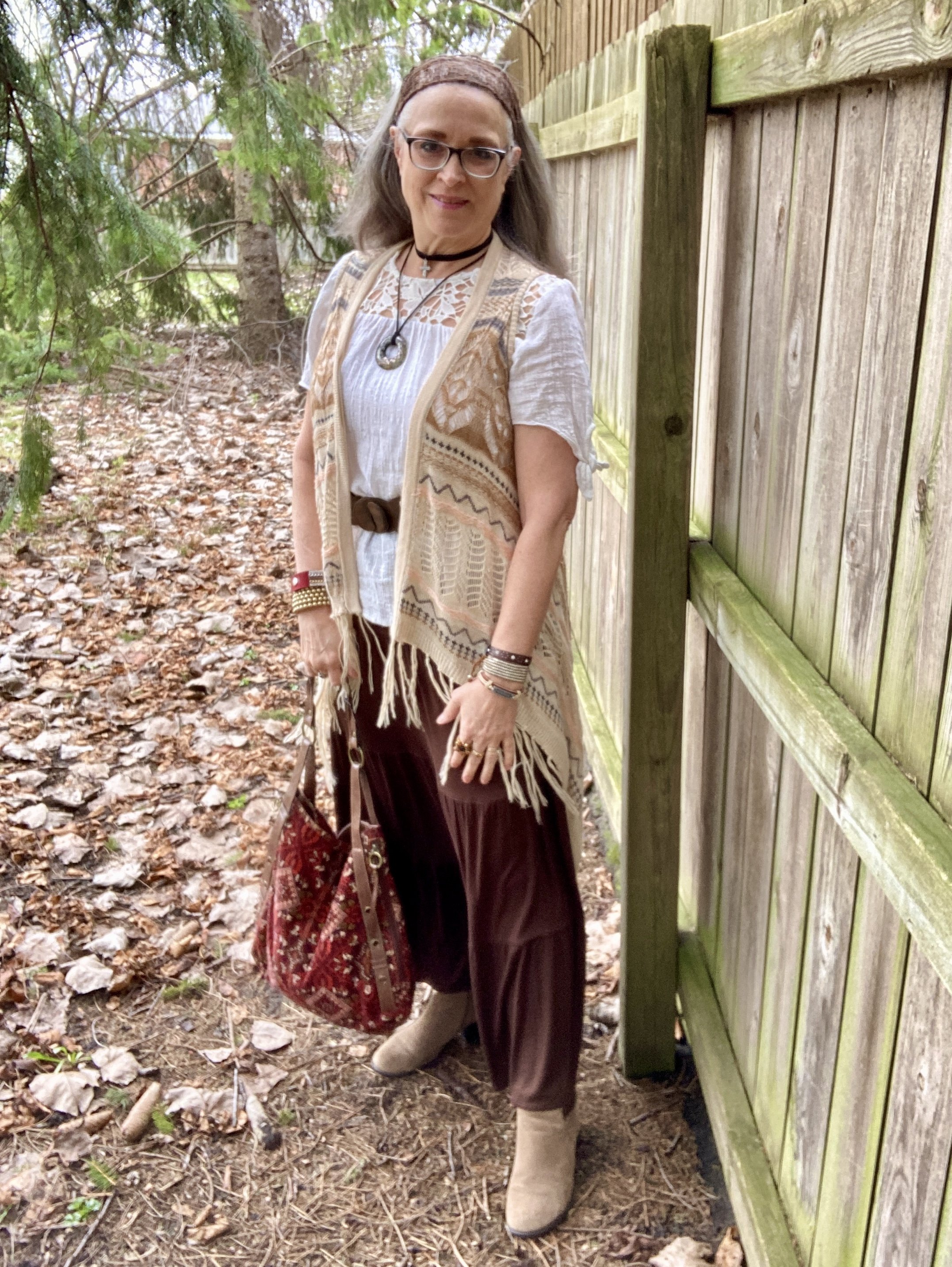A woman stands in the center of the image, set against a backdrop of scattered old pine tree needles and leaves, typical outdoor debris. She is standing in front of a weathered wooden fence on the right side, featuring three horizontal boards and a vertical post, with some planks tinged gray and green.

The woman is facing the camera, wearing black glasses and a headband that pulls her long hair back. She is dressed in a white blouse beneath a poncho-style vest that appears to be grayish or brown knitted material. A dark, champagne-colored skirt extends to her ankles, while she wears tan felt or suede boots.

Adorning her neck are two necklaces: a black choker with a cross pendant and a slightly longer necklace featuring a circular stone. Both wrists are decorated with multiple bracelets, some braided and others appearing to be leather bands. Her left hand holds a red purse.

The background features a few trees visible in the distance, completing this detailed scene of a woman captured in a serene outdoor setting.